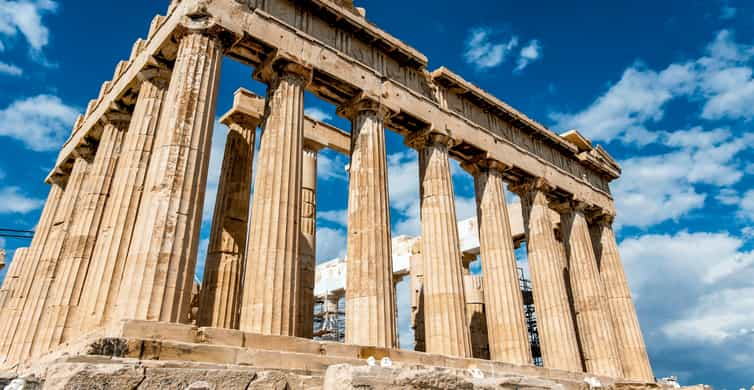This photograph vividly captures the crumbling grandeur of the Parthenon in Athens, Greece. At the foreground, three beige stone steps lead up to the ancient structure, setting a foundational stage for the ruins. A row of fluted columns, ranging in color from beige to light gray, stand prominently; eight columns are visible on the right side, with five additional columns discernible on the left. These majestic pillars, tapering upward, support a rectangular rim that is partially missing on the left but extends fully to the right.

Behind the primary row, a second layer of columns is partially visible, with two of these supporting a smaller beam of similar design. The structure exhibits significant wear, with pieces of stone crumbled away from both the top and the base, indicating its venerable age.

In the backdrop, a modest amount of scaffolding can be seen, hinting at ongoing efforts to preserve the edifice. The scene is set against a strikingly clear blue sky, adorned with puffy white clouds that flow across the horizon. The overall composition of the photograph highlights the timeless beauty and historical significance of the Parthenon, underlined by the serene and picturesque sky above.